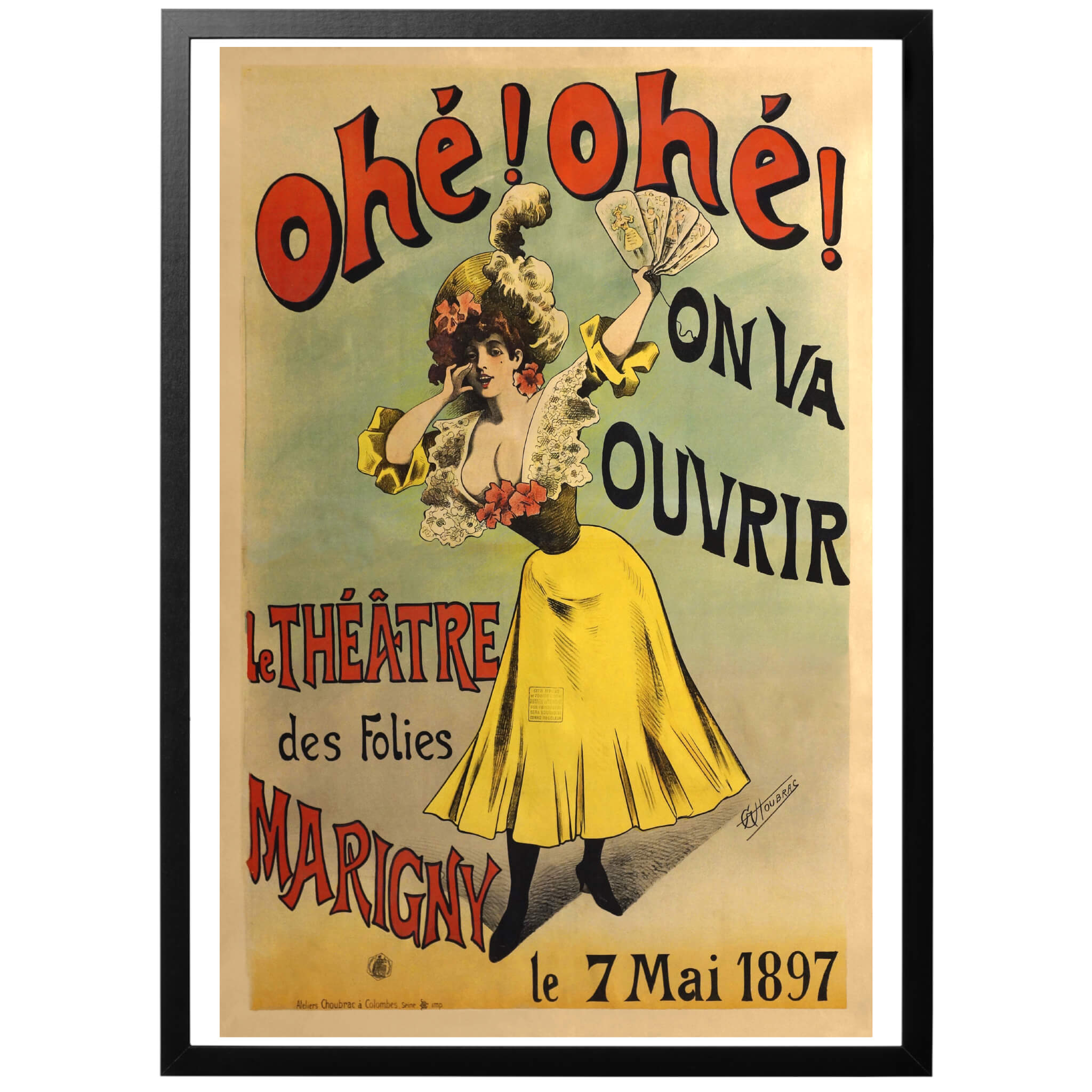This is an intricately detailed vintage French poster dated May 7, 1897, for a theater program at "Le Théâtre des Folies Marigny." Dominating the poster is a buxom woman who appears to be calling out to the viewer. She is elegantly adorned in a tight-fitting yellow dress, prominently accentuated with white and pink flowers, and complemented by a matching yellow hat adorned with similar floral designs. The dress features a corset, emphasizing her very tiny waist, and sleeves rolled up and ruffled. She holds a fan, contributing to her poised and alluring stance. The text elements are in bold red and black, with "OHE, OHE" prominently displayed at the top, and the date "Le 7 Mai 1897" in the bottom right corner. Additional text such as "Le Théâtre des Folies Marigny" appears on the left side, rendered in a striking red with a black outline. An artist's signature is also present in black at the bottom right corner. The overall aesthetic suggests the poster is an advertisement for a theatrical event, vividly capturing the elegance and allure of the era.